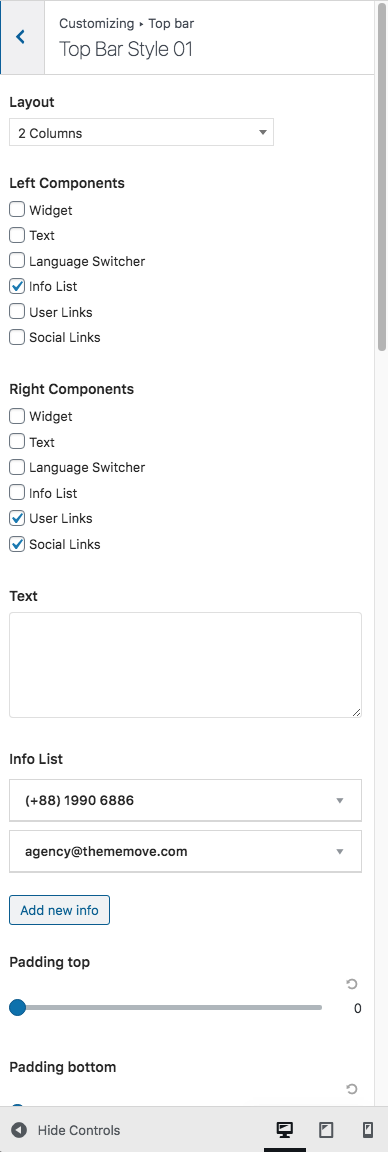The image showcases a menu interface for customizing the top bar's appearance on a white background. At the top, there is a blue back arrow, followed by the heading "Customizing: Top Bar - Top Bar Style 01" in bold text. Below, the "Layout" section appears in black off to the left, with a dropdown menu underneath set to "Two Columns."

The section titled "Left Components" lists six checkbox options: Widget, Text, Language Switcher, Info List (checked in blue), User Links, and Social Links.

Similarly, the "Right Components" section features identical checkbox options with blue checkmarks next to User Links and Social Links.

Following this, a "Text" section includes an empty text box, with an "Info List" section below that, containing two dropdowns—one showing "+8819906886," and another "agency@themove.com". A blue-outlined box labeled "Add New Info" follows these elements.

At the bottom, the "Padding Top" setting is adjusted via a slider bar, with a blue dot positioned to the left. Below this, "Padding Bottom" is listed without a visible adjustment mechanism. Finally, there are controls for different viewing modes: Hide Controls, Desktop Icon, Tablet Icon, and Phone Icon.